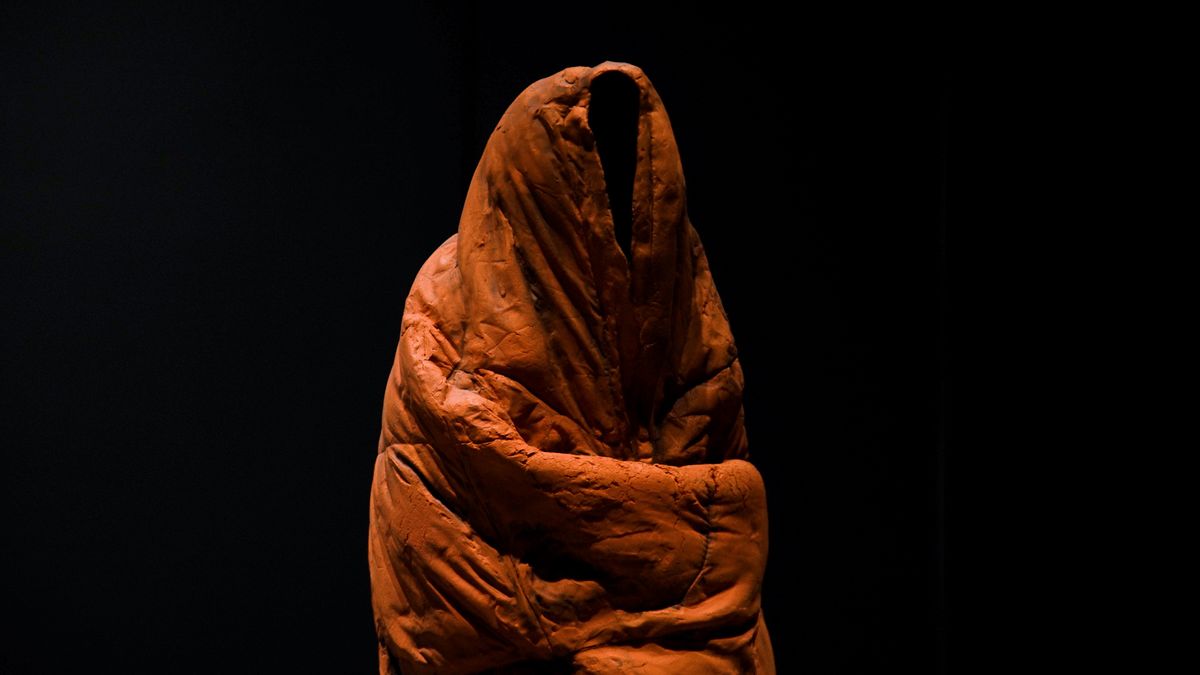In the mysterious photograph, a dark, uniformly black background serves as the stage for a curious focal point: a shape that resembles a person wrapped tightly in a quilt or comforter. The fabric, a dull burgundy with an occasional lighter red or rust hue where the light catches it, is marked with distinct stitching and numerous wrinkles. This gives the appearance of a figure sitting on a chair or stool, arms presumably crossed in front, creating a pronounced bulge that suggests an arm wrapped around the body. The top of this wrapping forms a triangular opening with a curved line that might indicate where a head would be, but this area is shrouded in pitch-black darkness, rendering any face invisible. Light appears to illuminate the scene from the left, enhancing the texture and folds of the fabric, yet leaving the opening in deep shadow, contributing to the overall enigmatic atmosphere of the image.